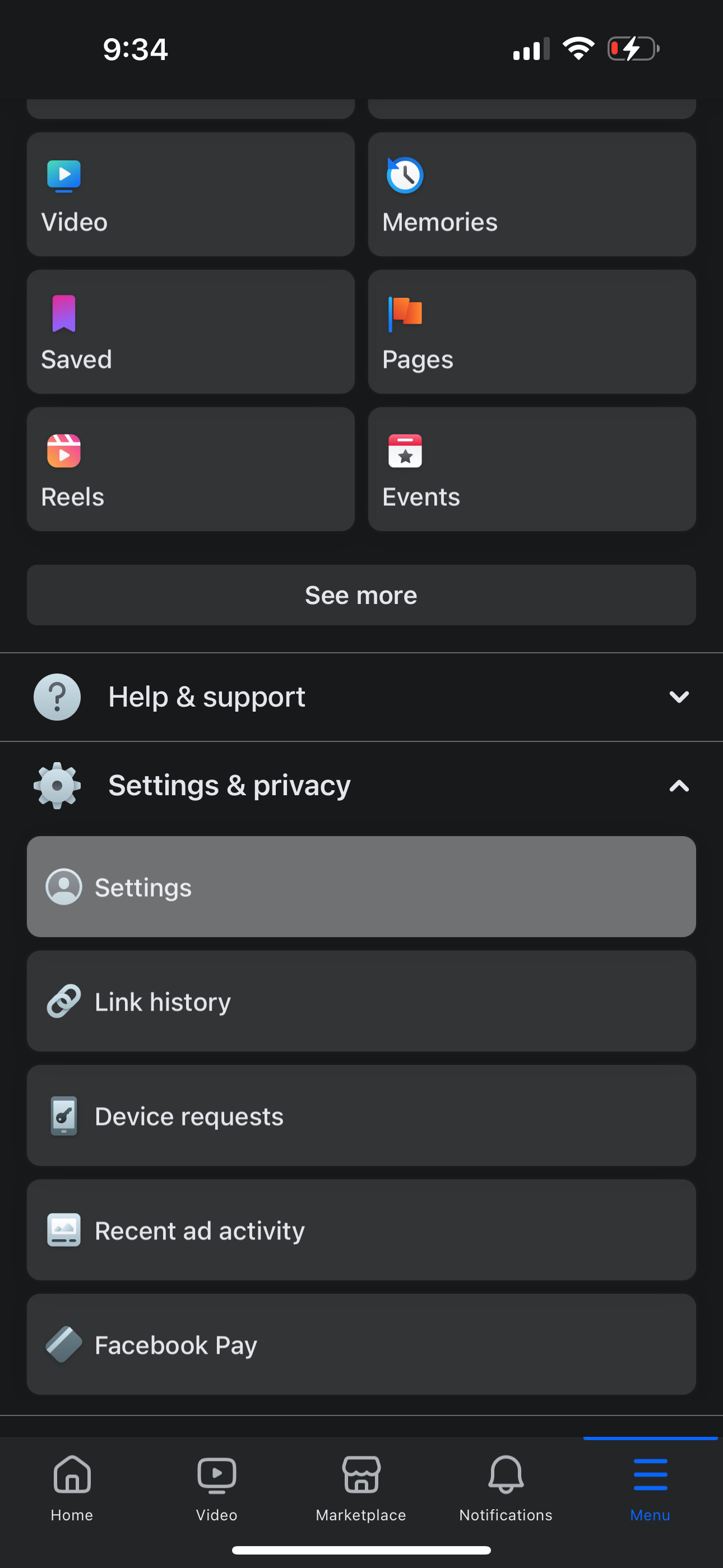This smartphone screenshot features a predominantly black background, highlighting a high degree of contrast. In the top-right corner, there is a timestamp reading 9:34, accompanied by a battery icon signaling a low battery with a red warning icon, and a Wi-Fi icon indicating a connected network.

The interface displays two columns of tabs, with the left column starting from the top with "Video," followed by "Saved," and at the bottom, "Reels." The right column, from top to bottom, includes "Memories," "Pages," and "Events."

Below these columns, a "See More" button appears, which expands additional options. Following this, a section marked with a question mark icon is labeled "Help and Support," with a dropdown arrow indicating expandable options. Another dropdown titled "Settings and Privacy" is expanded, revealing "Settings," which is currently highlighted.

Under "Settings," there is a link icon preceding the text "Link History." Further down, icons are paired with their respective texts: "Device Requests," "Recent Ad Activity," and "Facebook Pay."

At the very bottom of the screen are navigation buttons: a "Home" button, a "Video" button, a "Marketplace" button, a "Notifications" button, and a "Menu" hamburger button, arranged from left to right along the bottom border.